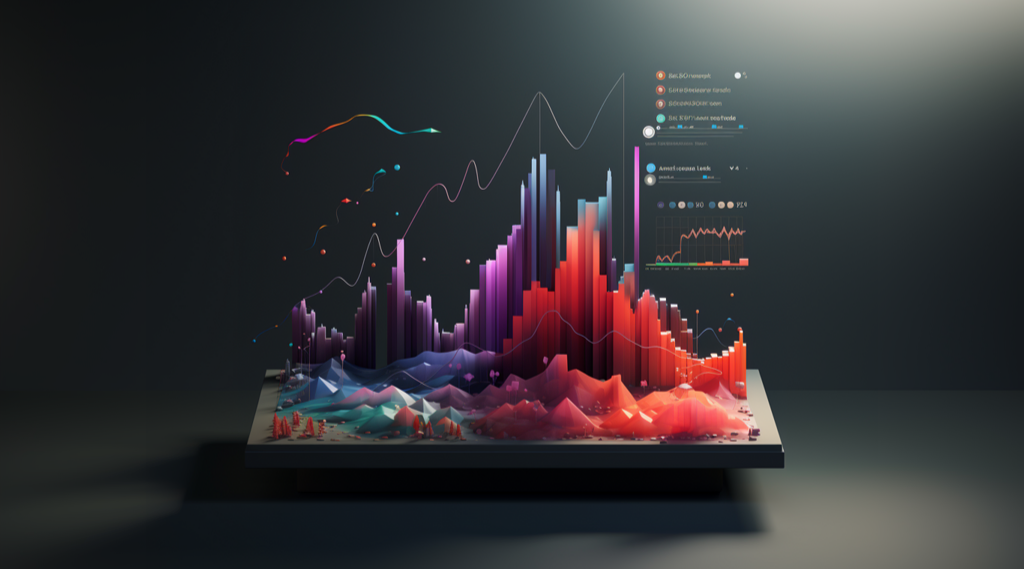In a dark, floating room, a gray platform supports an intricate, AI-generated, three-dimensional graph. The graph features an array of colorful elements: blue graphs positioned in the back, followed by purple ones in front, then red graphs, and at the base, there are mountainous, crystal-like structures rendered in vibrant hues of blue, turquoise, pink, and red. The platform appears to hover over a gray surface, illuminated by a light source from the top right that emphasizes the three-dimensional aspect of the scene. The perspective of the graph is slightly off, with the base appearing wider in the distance than in the foreground. To the right of this compelling visual, there is a partially blurred legend and semi-transparent data tables, detailing the various components but hard to decipher from a distance. The overall effect is a striking representation of a graph in a 3D space, seamlessly blending line and bar graphs with sculpted, rocky forms.